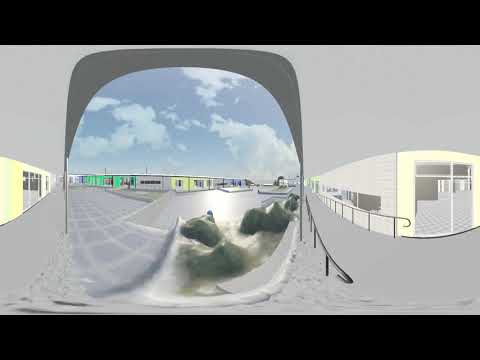The image depicts a surreal outdoor scene that appears to blend computer graphics and photography. At the forefront, there's a curious, distorted lens or rear-view mirror in the middle of the frame, providing a warped view of the surroundings. This central element showcases a fragmented view of a parking lot area, bordered by a gray railing that suggests an outdoor setting next to a building. Through this lens, one can see an expansive sky with light blue hues and fluffy white clouds, as well as distant buildings in varying colors, including yellow and mint green.

Beyond the distorted lens, the scene becomes more abstract and difficult to interpret, though it hints at a beachside or boardwalk area with sand near the dark railing. The buildings in the background appear as colorful, low-level one-story commercial or industrial structures, some with flat roofs and bay doors. The overall image, which might be an artistic composition or an animation, has an air of artificiality and abstraction, making real-world elements like the building's flat roofs and the surrounding outdoor area blend seamlessly into the surreal visual experience.